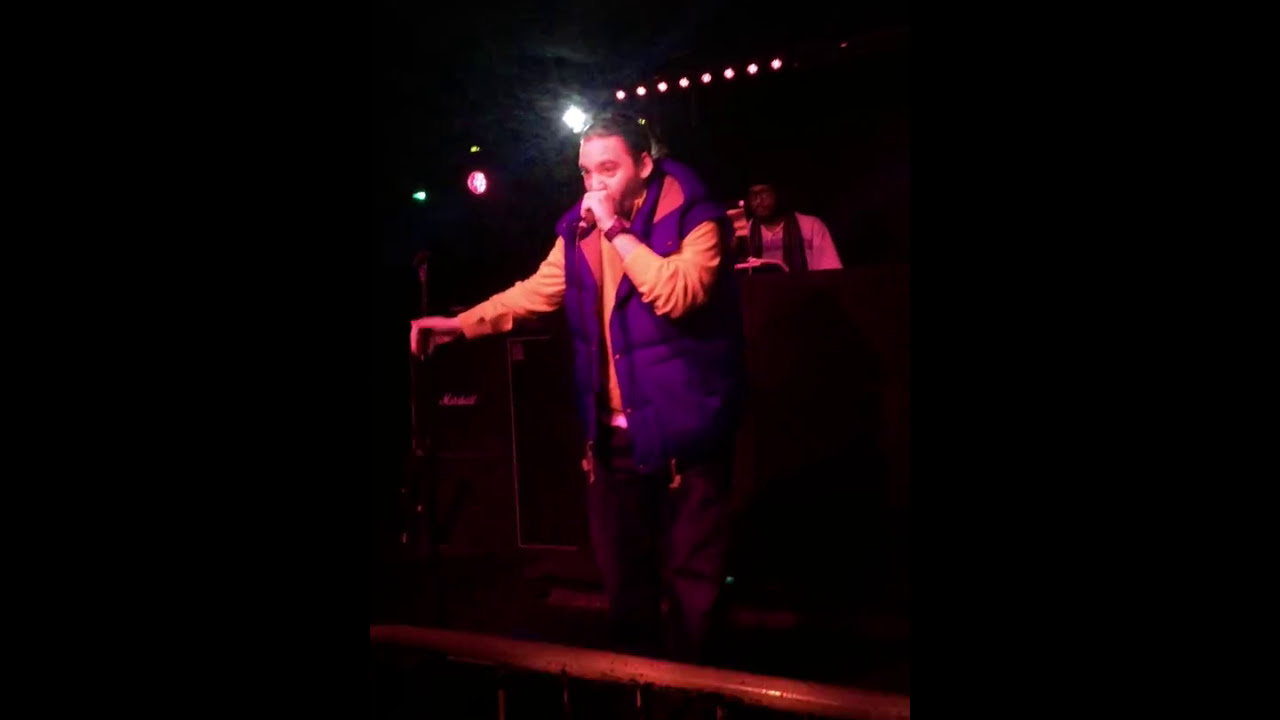In this dimly lit image, a man performing on a stage commands attention. He wears a vibrant ensemble consisting of an orange long-sleeve shirt layered with a purple vest. His dark hair frames his face as he holds a microphone to his mouth, poised in mid-speech or song. The stage itself, illuminated faintly, has a dark brown mahogany step beneath his feet. Above him, a row of lights creates a dramatic ambiance, with a notably bright light to the right and colorful lights to the left that evoke a concert atmosphere. His right arm is extended forward, adding dynamic movement to the scene. Behind him, partially obscured in the darkness, stands another figure in a white shirt with long black hair, possibly a DJ or backup performer, contributing to the depth and liveliness of the performance setting.